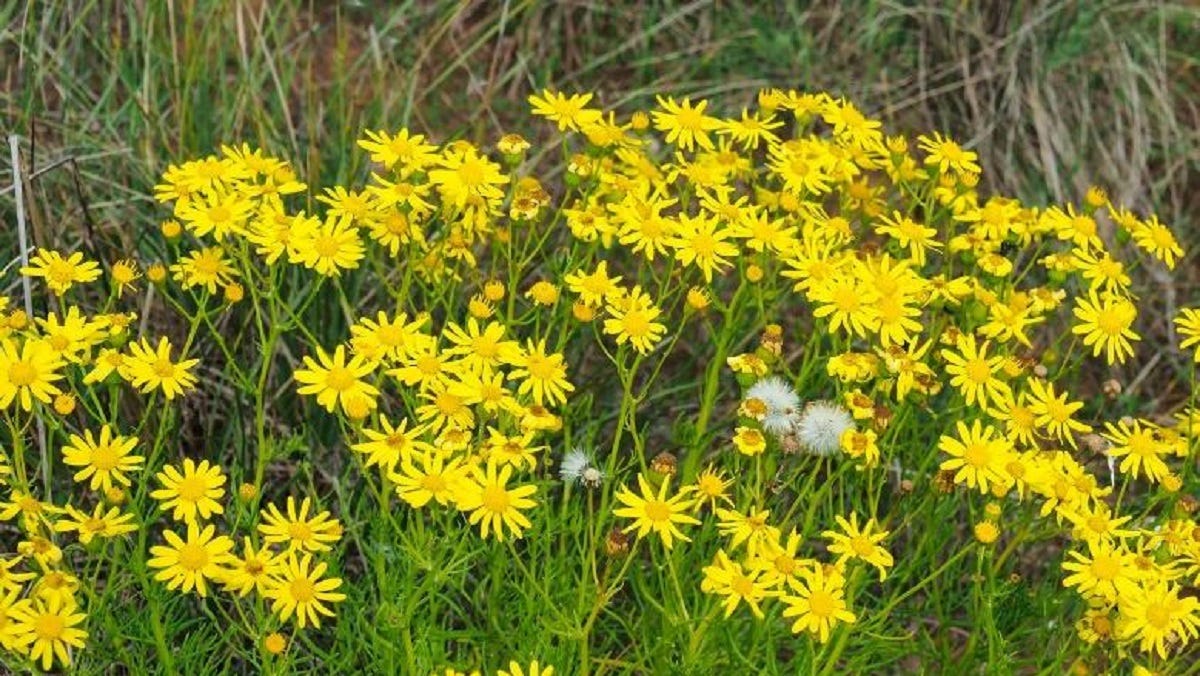This photograph captures a large patch of wild yellow flowers, likely dandelions, growing in a natural, weedy area. The scene is set in a horizontal, rectangular format with the flowers occupying around 80% of the frame. The vibrant yellow flowers, both blooming and turned into white puffballs, stand on thin green stems amidst tall, rough grass that's a mix of green and brown shades. The backdrop reveals more of this wild grass, suggesting a marshy or wooded area. The lighting appears subdued, possibly taken in the shade or on an overcast day, with no bright sunlight illuminating the scene. The image is text-free and human-free, with the primary colors being yellow, green, brown, and white.